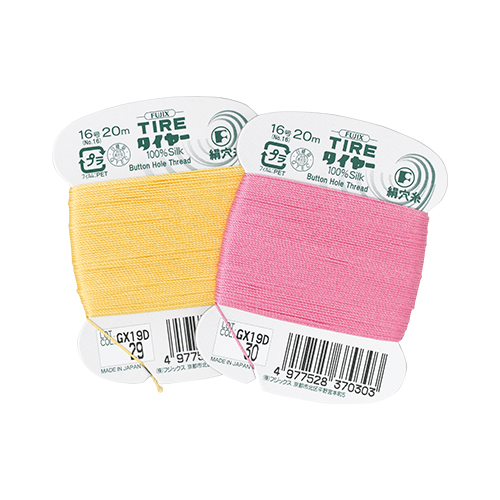The image features an up-close view of two spools of thread, each wound tightly around flat, white cardboard holders. The spool on the right, tilted diagonally to the right, contains soft pink thread, while the one on the left, slightly tilted to the left, holds soft yellow thread. Both cardboard holders display green text, including the brand name "TIRE" and the specifications "16 20 meters," along with "100% silk buttonhole thread." The holders also feature several logos and what appear to be Asian characters. At the bottom of each holder, a black and white UPC barcode is visible, alongside a lot number such as "GX19D-30." The entire setup is set against a pristine white background, highlighting the details and colors of the threads and their packaging.